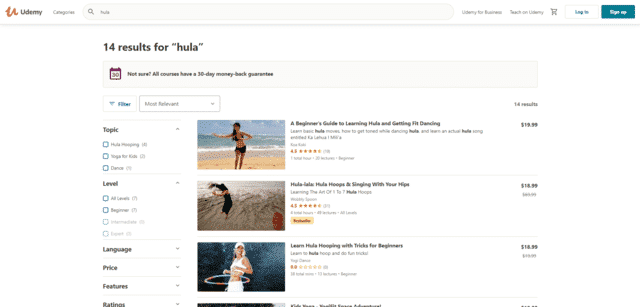The image depicts an online learning platform, Udemy, showcasing a search for "Hula" courses. At the top of the interface, the word "Udemy" is prominently displayed, followed by navigation elements including a magnifying glass icon within the search bar, a shopping cart symbol, a sign-in button, and an unidentified blue box. Below these elements, there is a notification stating "14 results for Hula."

The page also features several filter options, each with checkable boxes: Categories, Topic, Level, Languages, Price, Features, and Ratings. The text within these filters is too small to discern.

Moving down, the search results begin with the first course showing an image of women dancing, priced at $19.99. The second course features a woman on a beach, priced at $16.99—a detail that is hard to confirm due to the small font size. The third listing depicts a woman using a hula hoop, priced at $14.99. These courses all have accompanying text descriptions, though the font is too minuscule to read clearly against the white background. Each listing contains a concise visual representation of hula activities, primarily showcasing women engaged in dancing and hula hoop exercises.